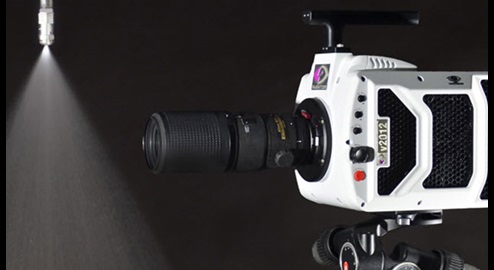This detailed color photograph showcases an industrial-type camera positioned on the right side of the image, facing left. The camera boasts a stark white casing with the model number "V2012" inscribed on its side. Dominating the scene is the camera's notably long black lens, which extends to the middle of the frame. The top of the camera features a gray bar with five buttons aligned vertically; four are black buttons, while the bottom one stands out in red.

Mounted on a stand that can raise or lower, the camera commands attention against a solid black background. To the top left corner of the image, a light fixture—sometimes mistaken for a sprinkler—casts a prominent beam of light downwards, illuminating the scene. An additional detail is a logo on the front of the camera comprising black, gray, and purple elements. The composition is meticulous, highlighting both the functional and aesthetic elements of the camera in sharp, clear detail.